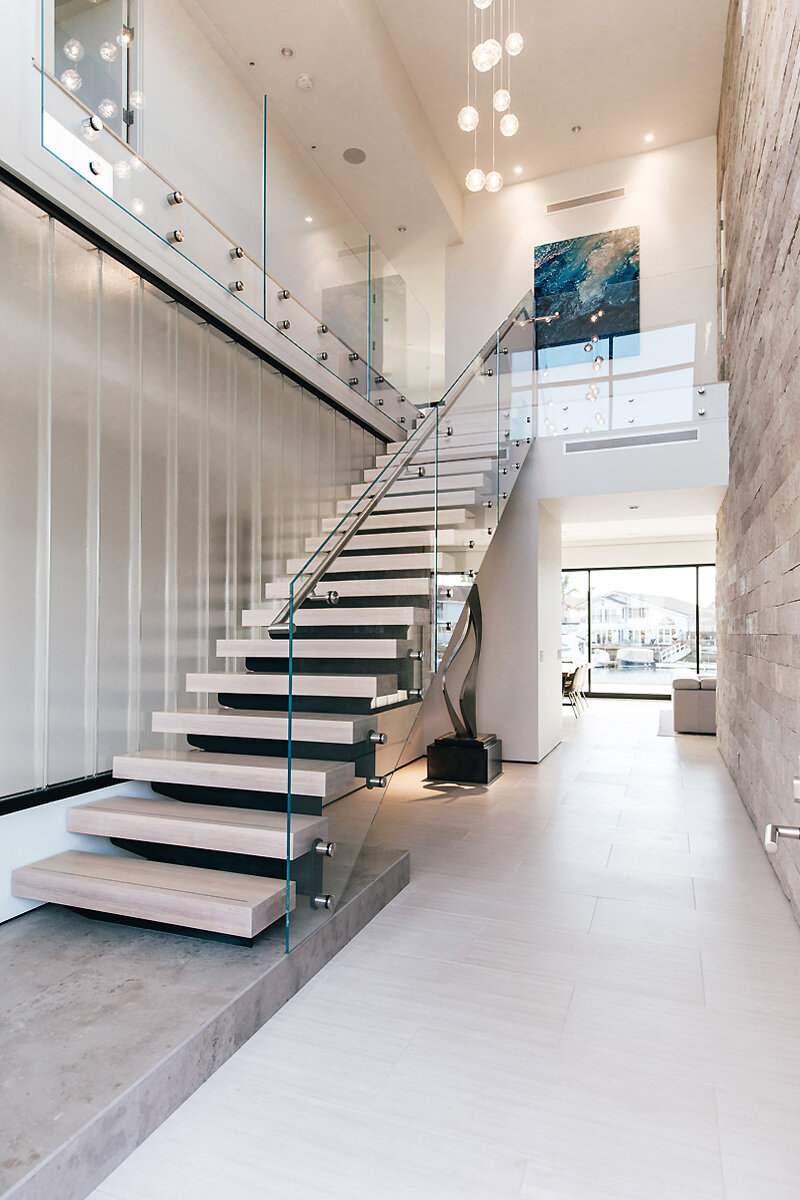This photograph captures the interior of a spacious and modern home. The central feature is a staircase on the left, ascending to an upper level. The stairs and balcony above boast sleek, transparent glass railings, emphasizing the home's contemporary design. A stone wall on the right adds texture and complements the predominantly white and beige color palette. Art adds a splash of color, including a notable blue painting on the landing. The floors, a pristine white tile, further enhance the bright and airy feel, accentuated by abundant natural light streaming through large, floor-to-ceiling windows. Beyond these windows, one can glimpse another house across the street, nestled beside a dock with ramps and boats. The ceiling features elegant, dangling light fixtures, which illuminate the space in a soft, inviting glow.